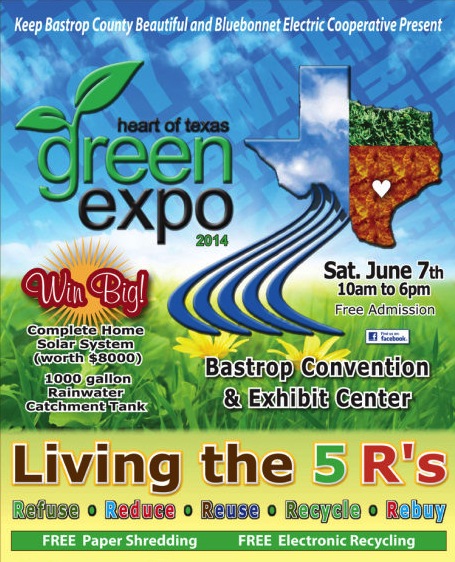This is a vibrant and detailed poster for the Heart of Texas Green Expo 2014, organized by Keep Bastrop County Beautiful and Blue Bonnet Electric Cooperative. The event is held on Saturday, June 7th, from 10 a.m. to 6 p.m. with free admission at the Bastrop Convention and Exhibit Center. The background of the poster features a lush grassy field with yellow flowers and a clear blue sky, giving it a refreshing and eco-friendly feel. Dominating the image is a notable graphic of the state of Texas, segmented into blue, green, and brown areas with wavy lines, and a bright sun graphic that highlights the "Win Big" slogan. The main attractions include a chance to win a complete home solar system worth $8,000 and a 1,000 gallon rainwater catchment tank. The event promotes the slogan "Living the 5 R's: Refuse, Reduce, Reuse, Recycle, Rebuy," and offers free paper shredding and electronic recycling. The poster also features a Facebook logo to connect people to more event updates.